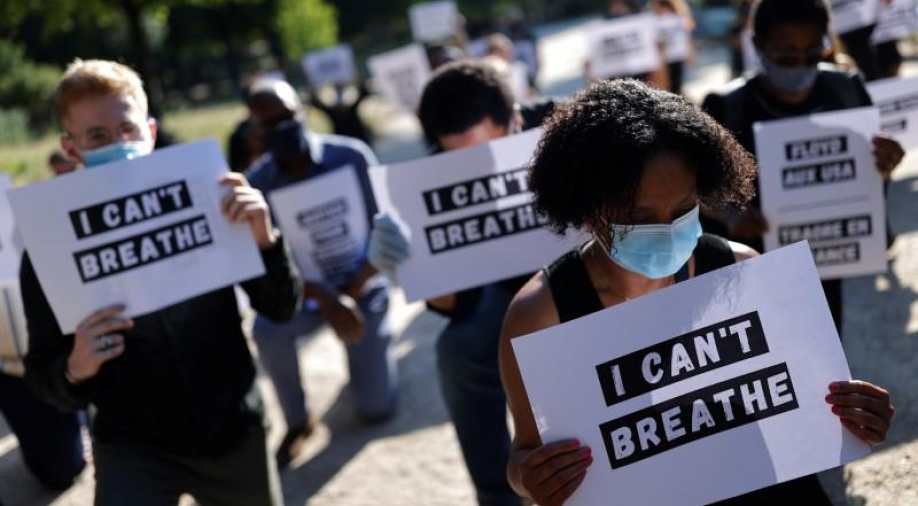The image captures a protest related to the George Floyd murder, showcasing a diverse group of individuals gathered in solidarity. The focus is on a few prominent figures in the forefront: a Caucasian man with short blonde hair and glasses, and an African-American woman with curly black hair. Both are wearing masks, as are the other protestors surrounding them. Everyone is holding signs printed on white paper with bold black text, featuring the phrase "I can't breathe"—the "I can't" in white lettering on a black background, with "breathe" below in black lettering on white. The image, though somewhat blurry towards the back, clearly shows participants both standing and kneeling. The setting appears to be a public area with sand or gravel underfoot, and trees and grass visible in the background. Some signs have additional text, including references to Floyd, AUX, and USA, albeit less legible. The scene powerfully captures the unity and determination of the protestors amidst the backdrop of a peaceful protest.